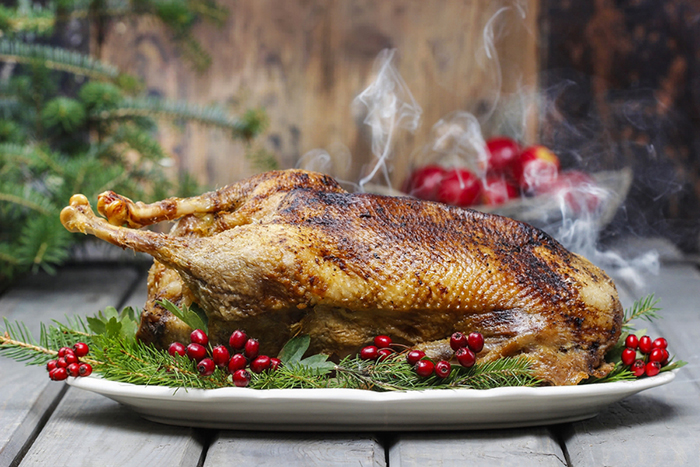A beautifully detailed image showcases a large, perfectly roasted chicken, or possibly a goose, resting on a long white plate. The plate sits on a slatted gray table, possibly a patio area, featuring a delightful arrangement of festive decorations. Surrounding the roasted bird are pine tree needles adorned with red berries, reminiscent of holly. Steam rises enticingly from the dish, filling the air with a mouthwatering aroma. In the upper left background, there is a hint of green pine and a blurred wooden wall. Further back, a bowl brimming with red and yellow apples adds a splash of vibrant color to the scene. The presentation is exquisite, making the dish look exceptionally appetizing.